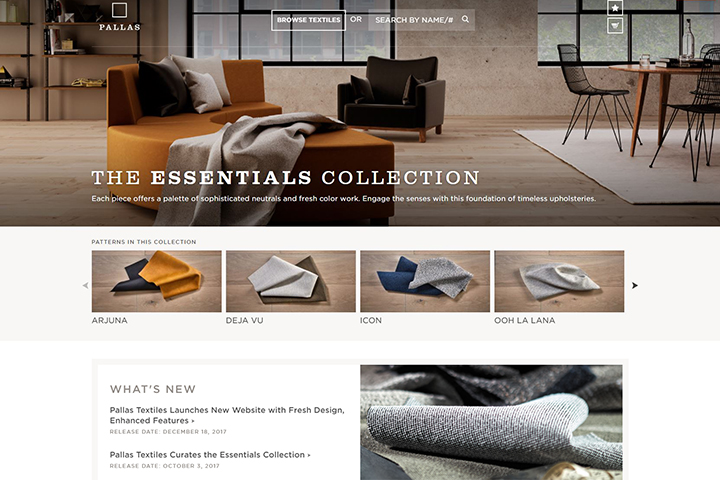The photograph captures a cozy and inviting interior of a home featuring a warm wooden floor. Centered in the room is a comfortable sofa accompanied by a stylish chair and a well-crafted wooden table. Two large windows provide natural light, with one revealing the view of a neighboring brick building, and the other offering a scenic outlook of lush trees.

On closer inspection, the image contains an overlay of a web page for Pallas Textiles. Positioned above the tree-view window, the webpage showcases various elements. There is a search bar at the top with the text "Search by name" inside it. Nearby, two square icons—one depicting a star and the other a shopping cart—enhance user navigation. 

The content of the website focuses on Pallas Textiles' "Essentials Collection," described as offering a sophisticated palette of neutrals and fresh colors, designed to engage the senses with timeless upholsteries. Patterns highlighted within this collection include "Arjuna," "Deja Vu," "Icon," and "Ooh La Lena."

Additionally, the website announces new updates: "What's New" features the launch of a redesigned website with enhanced features, dated December 18, 2017. Another announcement details the curation of the Essentials Collection, with a release date of October 3, 2017.

This detailed description captures not only the cozy ambiance of the home’s interior but also the textured, informative overlay of the Pallas Textiles website.